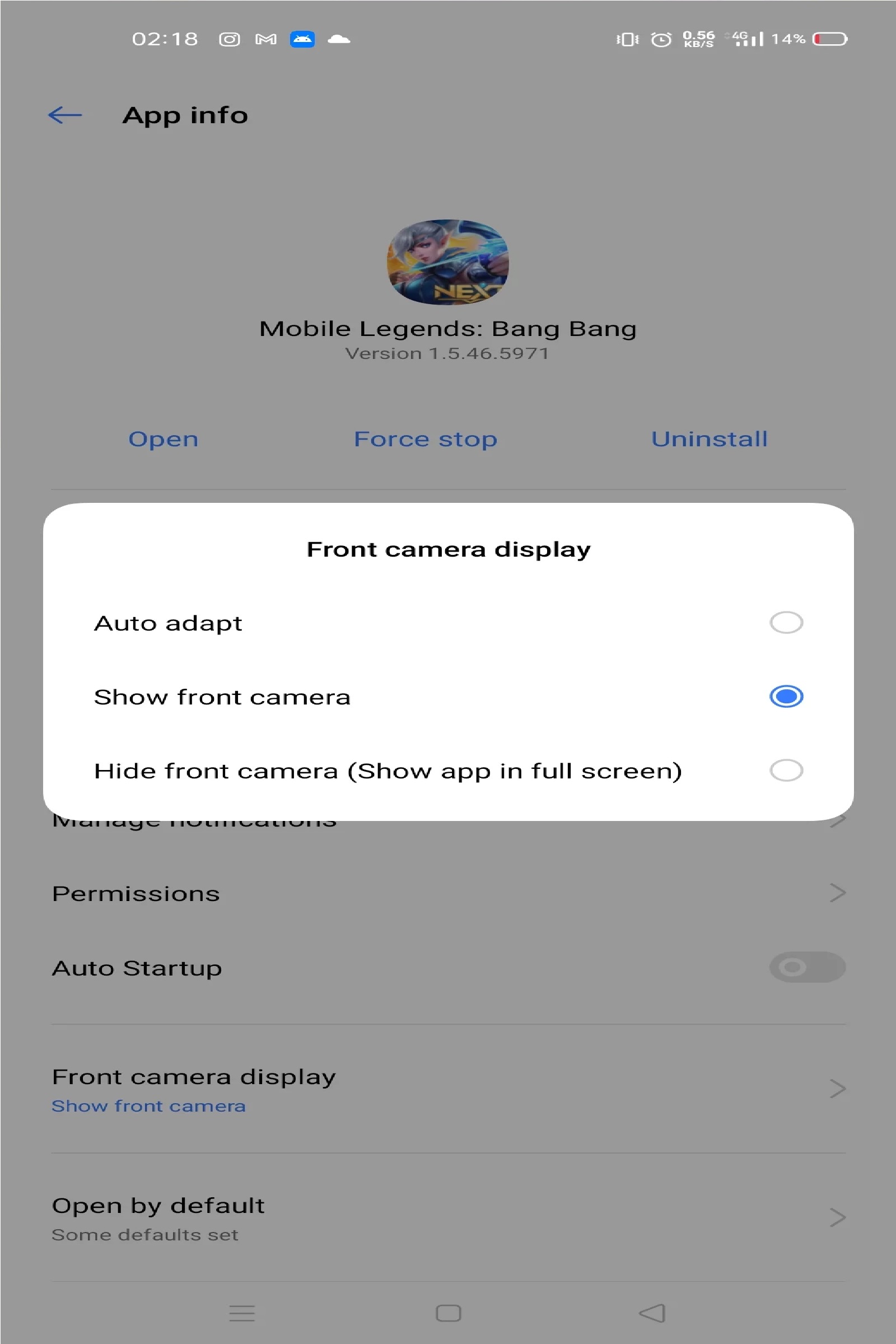The image is a screenshot from a cell phone display. The background is predominantly gray, with a white rectangle taking center stage. Beginning at the top of the image, the time reads "2:18 PM," and a series of icons are visible, including a battery icon in red, indicating that the phone needs to be charged. 

Within the white rectangle, there is a blue arrow icon positioned next to the text "App Info." Below this, there’s a cartoonish illustration with the partial text "NEX" and an animated character who appears humanoid with white hair. This character is depicted holding a laser beam. The text "Mobile Legends: Bang Bang" is clearly visible, followed by the version specifics of the app.

Further down, the text "Front Camera Display" is displayed prominently. To the left, there's an option labeled "Auto Adapt" with an adjacent clickable circle, which is not selected. The text "Show Front Camera" is present with a circle next to it, which is marked, indicating it is selected. At the bottom, there is an option labeled "Hide Front Camera (Show App in Full Screen)," which remains unchecked.